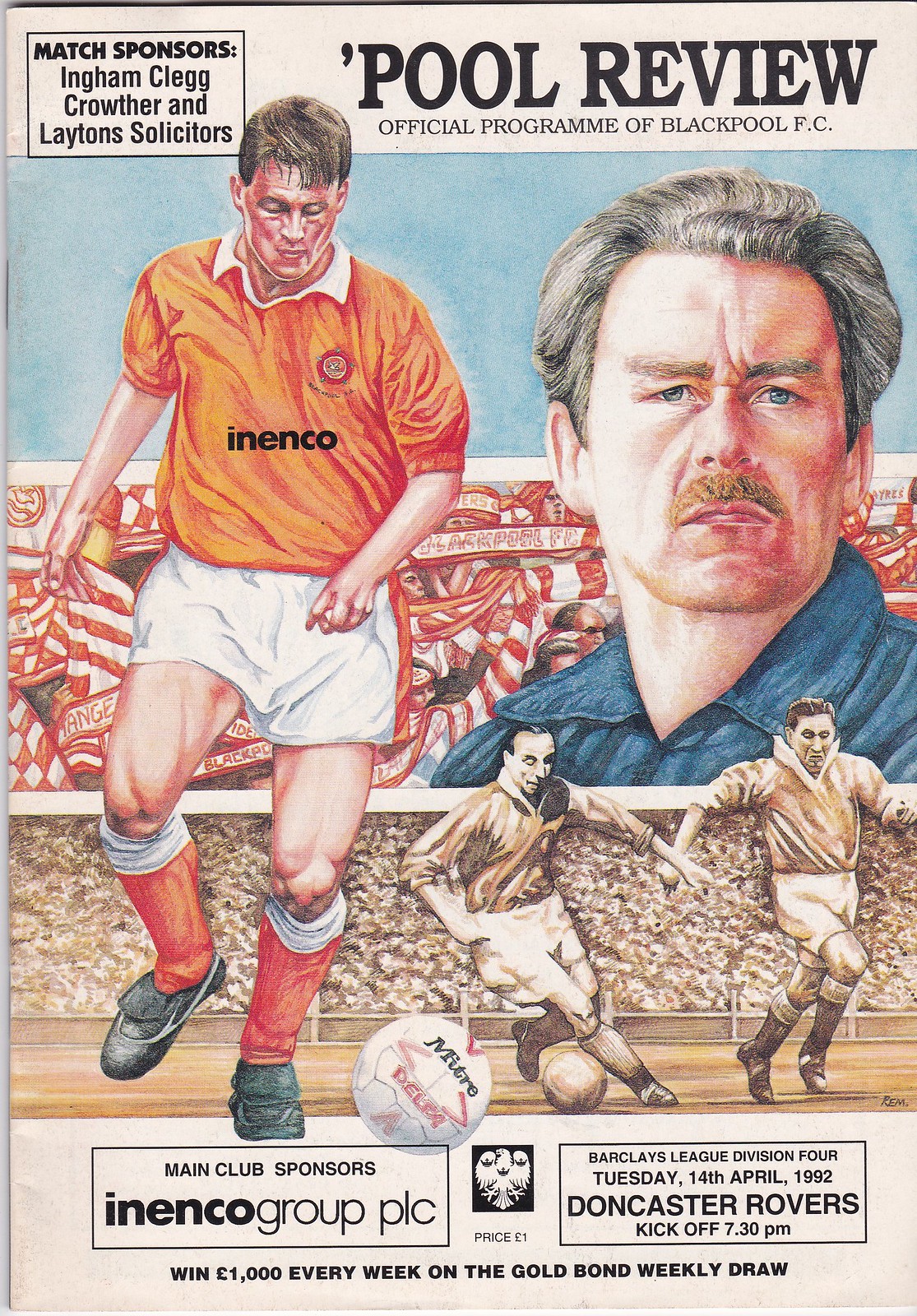The rectangular image is the cover of an official program for Blackpool FC, titled "Pool Review." On the top left, a black box contains the match sponsors, "Ingham Clegg, Crowther, and Leighton Solicitors." The primary illustration features a soccer player in mid-play, wearing an orange jersey with "INENCO" written in black lowercase letters, white shorts, and orange socks. He is chasing a soccer ball. To the right, there is a separate illustration of a man, likely a coach, with a mustache, wearing a dark blue collared shirt and sporting a serious expression. Beneath him, another illustration depicts two players in black and white, also in mid-play, with a crowd visible in the stands behind them.

Across the bottom of the cover, two outlined rectangles contain additional information. The left rectangle states, "Main Club Sponsors: INENCO Group PLC," while the right rectangle lists the match details – "Barclays League Division 4, Tuesday 14th April 1992, Doncaster Rovers, kickoff 7:30 p.m." In between these rectangles, there is a logo resembling three birds together, and underneath it is the price, "£1." At the very bottom, in small black text, it reads, "Win £1,000 every week on the Gold Bond Weekly Draw."